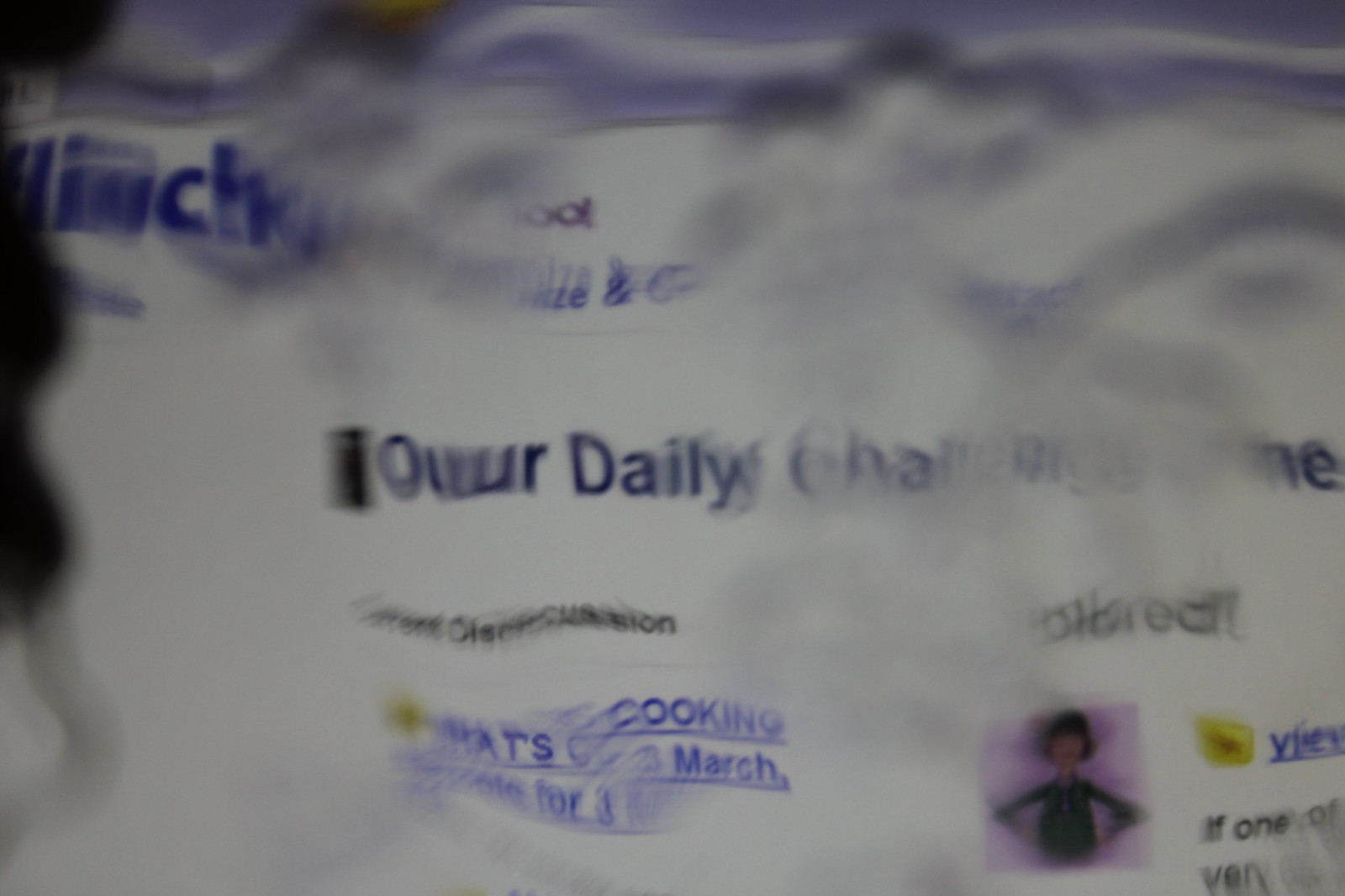The image is a wavy, blurry picture that appears to have been warped by a filter, giving it a smudged and distorted appearance reminiscent of looking through water-covered glasses. The background is predominantly white with streaks of greyish tones. It features textual elements in both black and blue colors, but much of the text is unreadable due to the distortion. Some of the decipherable text includes words like "hour," "cook," "march," and fragmented parts like "H," "I," "U," "CH," "OD," "Our Daily," and "hats."

The top left of the image contains a medium blue text, possibly serving as a header for what seems to be a webpage or a digital display, perhaps indicating a daily challenge or fitness site. Central to the image, more blue text is present, likely related to the content of the page, with additional blue text lower on the left side suggesting a hyperlink. The bottom right corner features a cartoon drawing of a human figure, potentially a woman, with her hands on her hips, possibly serving as an icon or user avatar. Overall, despite the heavy smudging and wavy effect, the image portrays a mix of textual information and a cartoon graphic against a predominantly white background.